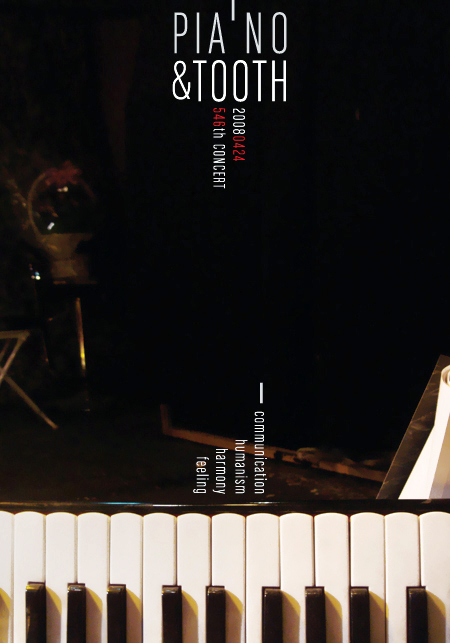This image is a detailed poster advertising a concert titled "Piano and Tooth." The top portion of the poster features a black background with some indistinct, dark designs, possibly including a chair and a rounded object on a table. Prominently, a row of piano keys spans across the upper section of the image, with the white keys at the top and the black keys at the bottom. The title "Piano and Tooth" appears vertically in the center. Below the title, horizontally, are the numbers "2008 04 24" with "04" and "24" in red, followed by "546th concert," also in red. At the bottom of the poster, vertical text lists the words "communication, humanism, harmony, and feeling." The overall design includes a shiny element, possibly resembling glass, and a white line separating the text from the lower section where the piano keys are prominently displayed.